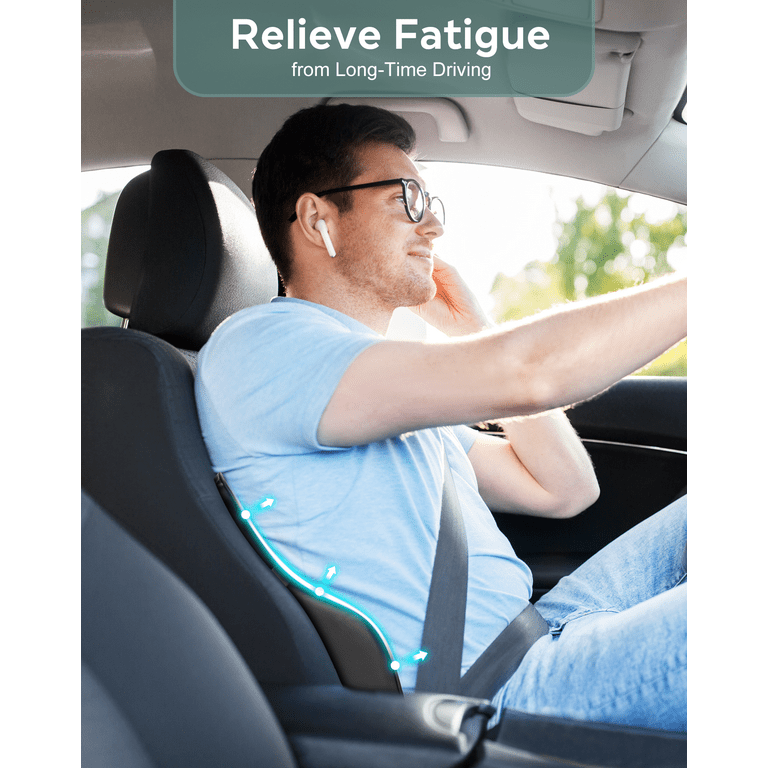The image depicts a man sitting in the driver's seat of a car, seemingly part of an advertisement aimed at promoting a backrest designed to relieve fatigue from long-term driving. The man, who appears to be Caucasian, has short brown hair and is wearing thick, round-framed glasses. He is dressed in a light blue t-shirt and blue jeans, with a gray seatbelt fastened over him. In his right ear, he wears an Apple AirPod. The car's interior features various shades of gray, with a darker gray driver's seat and a very light gray roof. The daytime sky is visible through the window, suggesting the photo was taken during the day. A neon blue line, accompanied by three dots and arrows, curves along the man's back, highlighting the ergonomic support provided by the backrest. At the top of the image, a semi-transparent green color block contains white text that reads, "Relieve fatigue from long-time driving."